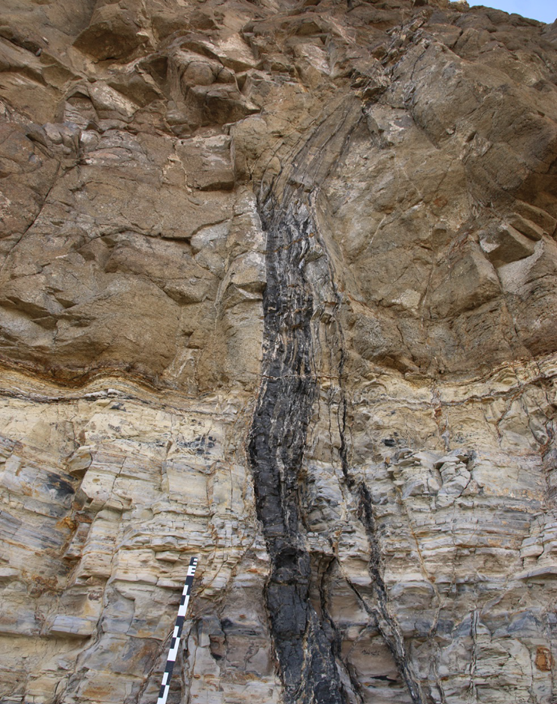This close-up photograph captures the rugged side of a mountain rock formation, predominantly featuring shades of brown that transition from tan at the bottom to darker hues towards the top. The image is tightly cropped such that both the base and the summit of the mountain are out of view, adding a sense of enormity to the cliffside which almost entirely fills the frame. Near the top-right corner, a small sliver of bright blue sky peeks through, contrasting sharply against the earthy tones. Dominating the center of the image is a prominent dark streak, resembling black goo or sludge, which appears wet and slick as it extends from the bottom upwards, fading as it reaches about three-quarters of the way up. Below the streak, more towards the left but still centrally positioned at the bottom, a black and white printed pole leans against the rocky surface. The rich texture of the rock, with its ridges and varied surfaces, is vividly detailed, conveying the precarious and raw beauty of the formation.